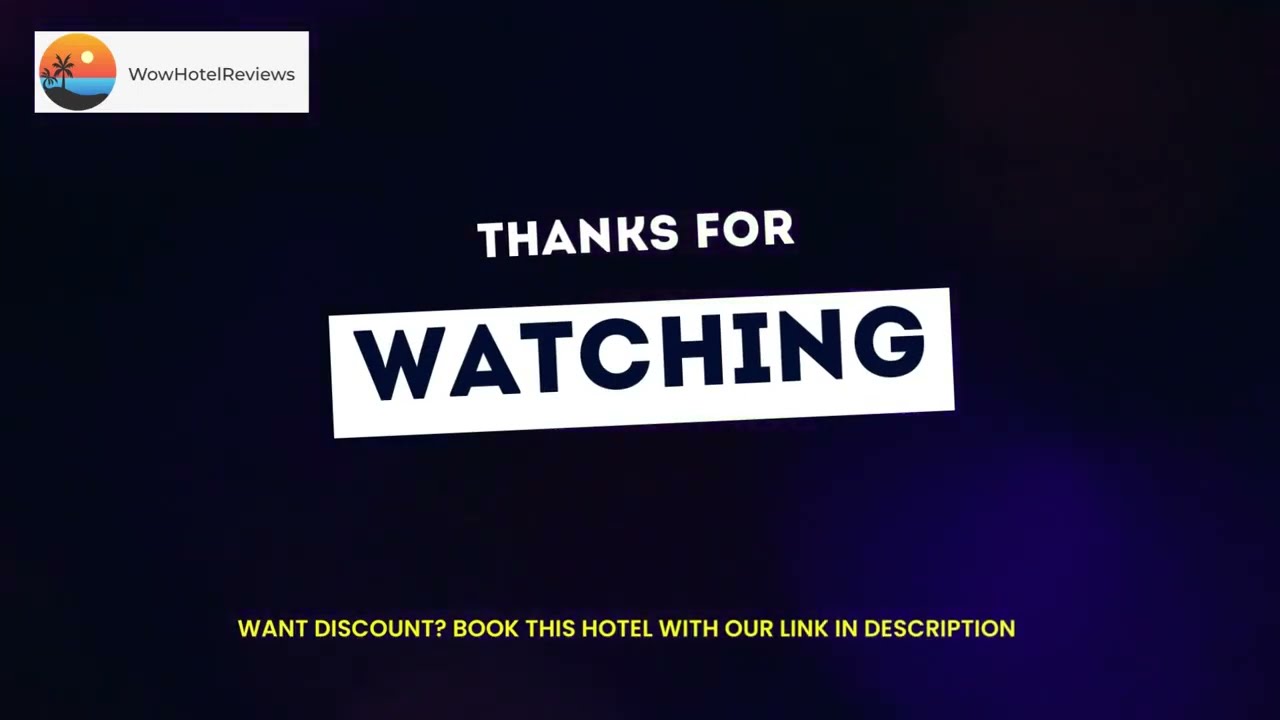The image features a text-centric design on a gradient background transitioning from dark black to navy blue, with the darkest area in the bottom right corner. In the top left, there is a white rectangle containing the text "Wow Hotel Reviews" alongside a circular logo depicting palm trees, an ocean, and a setting sun against an orange sky with green grass. Centrally positioned, large, white text reading "Thanks for watching" is outlined in blue, blending with the background. At the bottom, in yellow text, the message reads, "Want discount? Book this hotel with our link in description." This layout suggests it is likely an end screen for a YouTube video from the channel "Wow Hotel Reviews," encouraging viewers to book hotels through their provided affiliate links for discounts.